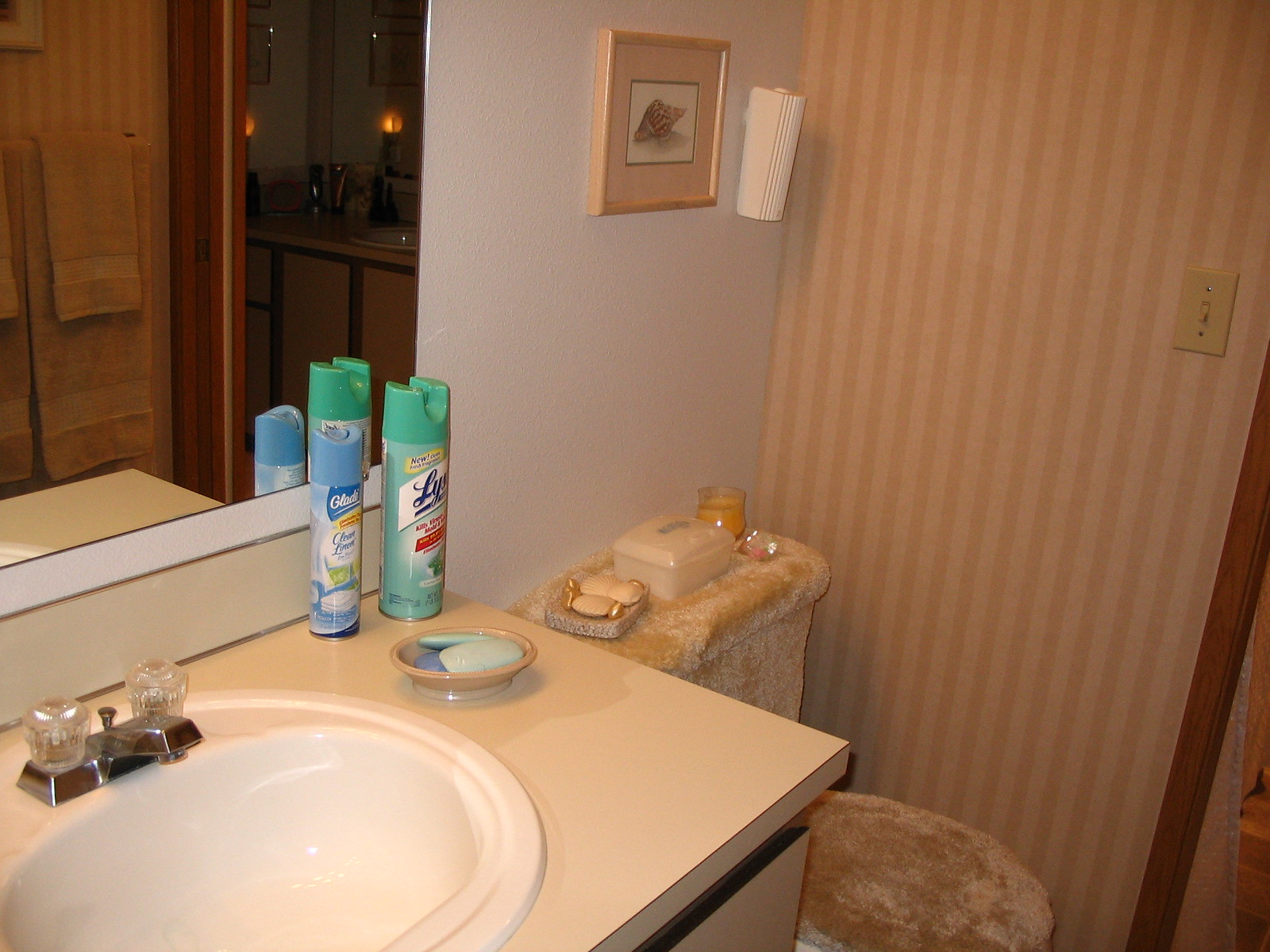This is a photograph of a meticulously clean residential bathroom showcasing a harmonious blend of beige and white tones with wood accents. The far wall features elegant striped wallpaper in shades of darker and lighter beige, complementing the room's overall decor. A white wall adorned with wood trim hosts a framed picture of a conch shell positioned above the toilet. The toilet itself is dressed in a cozy, furry seat cover and a matching tank cover.

On top of the toilet tank sit several decorative items, including a soap dish holder with neatly arranged soaps, two wet toilet paper wipes, and a yellow candle. To the left of the toilet, a sink with laminate countertops houses a white bowl sink, adorned with crystal knobs and a silver faucet. A soap dish to the right of the sink holds three pieces of blue bar soap, varying in shades of light blue, turquoise blue, and periwinkle blue.

The sink area also features two cleaning products: a blue-capped Glade Clean Linen air freshener spray and a turquoise-capped green Lysol spray. In the background, a mirror reflects another sink area and a set of yellow towels hanging against the yellow and beige striped wallpaper, adding depth and continuity to the room's design.